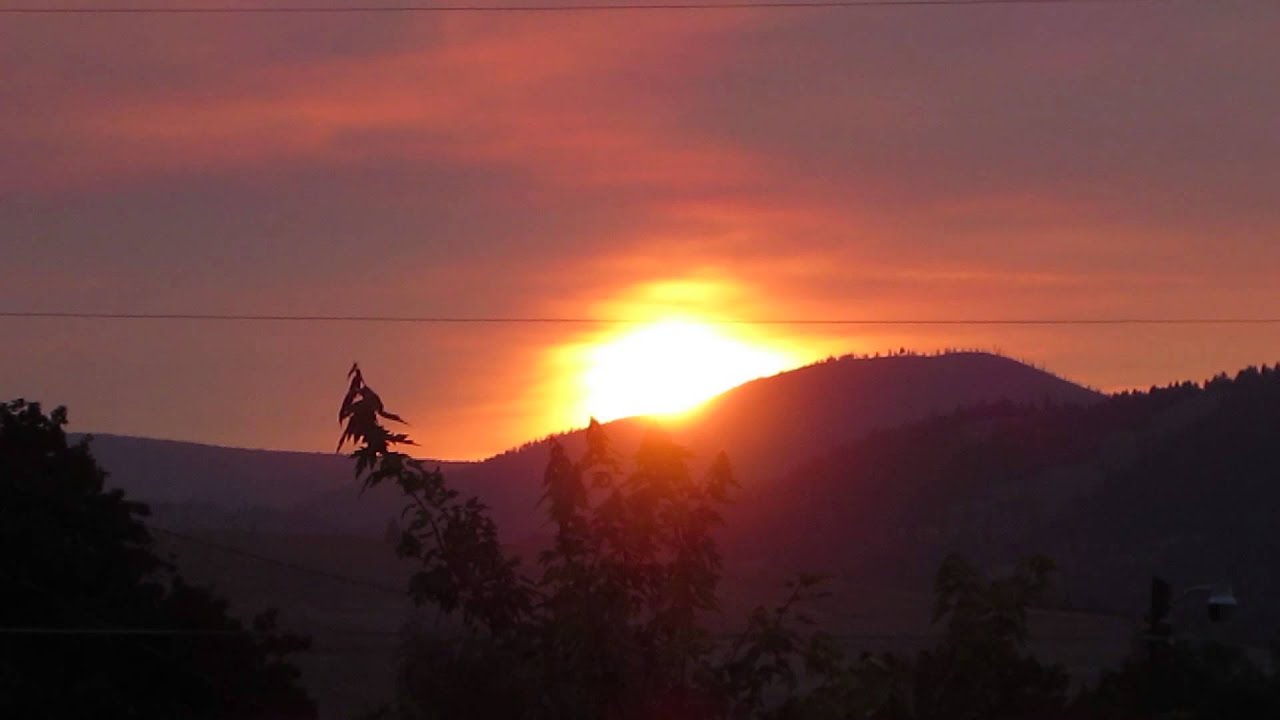A beautifully serene sunset showcases a partially hidden golden sun setting behind softly contoured hills, casting an enchanting glow that radiates warmth. The sky, adorned with rich and dreamy hues of orange, yellow, and pink, offers a striking visual contrast against the silhouetted dark shapes of the hills and the delicate outlines of plants or trees in the left corner. A thin wire runs horizontally across the scene, subtly intersecting the natural beauty. The image captures a tranquil moment where the sun's effervescent light dissolves into an ambient haze, creating an inspiring and peaceful tableau of nature.